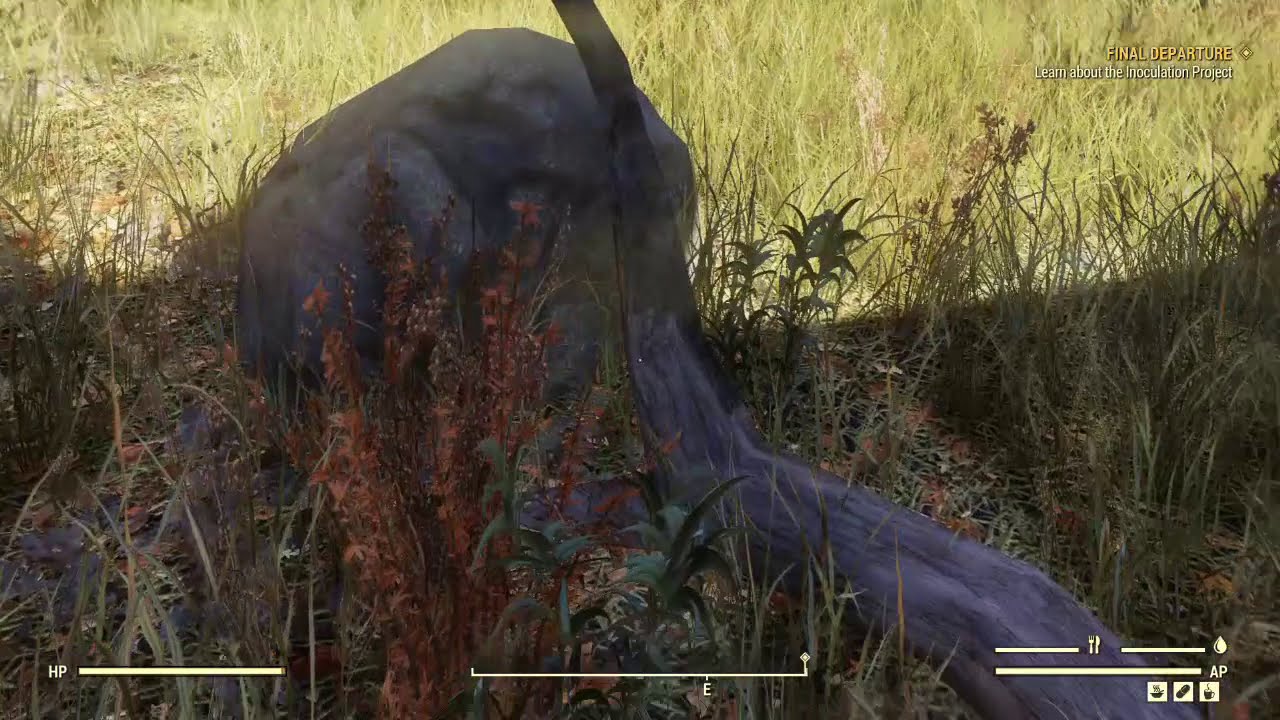This image appears to be a highly realistic digital rendering from a video game, showcasing an outdoor scene with a piece of wood leaning against a gray rock amidst lush green grass. The scene is richly detailed with earth tones, featuring purple and orange flowers scattered in the foreground and sunlight illuminating the upper half while the lower portion remains shadowed. The overall quality of the animation is almost photorealistic, though slight pixelation suggests its digital nature.

Text elements are dispersed throughout the image: in the upper right corner, yellow letters spell "Final Departure" with additional white text below reading "Learn About the Inoculation Project" accompanied by a plus sign. The bottom portion of the image features a Heads-Up Display (HUD) with several indicators. On the left, there is an HP bar, a thinner bar with an "E" in the middle, and on the right, a fork and knife symbol with lines and the letters "AP" alongside the icons, suggesting elements related to character health and survival mechanics.

The vivid depiction of the grass, wood, and rock combined with the sunlight and shadow effects, along with the intricate HUD elements, convey a scene that is both engaging and immersive, characteristic of a survival video game environment.